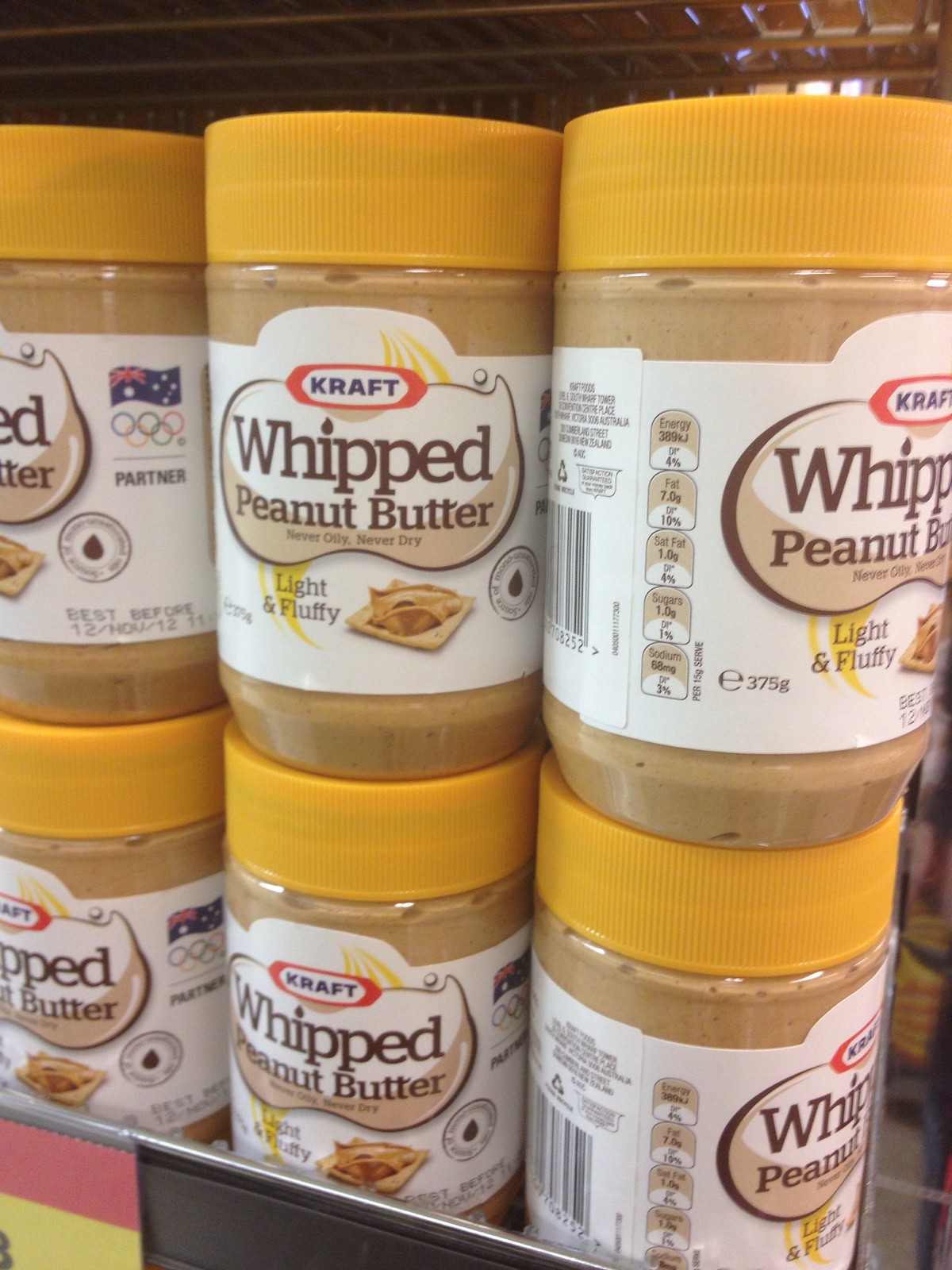This close-up image captures a store shelf stocked with six jars of Kraft Whipped Peanut Butter, arranged in two rows of three. The jars feature a yellow-orangey lid and a white label emblazoned with the Kraft logo. The label reads "Whipped Peanut Butter, Light and Fluffy," and includes a visual of a cracker topped with a dollop of peanut butter. Nutritional information such as fat content, saturated fat, sugars, sodium, and energy can be seen on some of the turned labels. Each jar has a net weight of 375 grams. Notably, the labels also display the Olympic logo and the British flag.